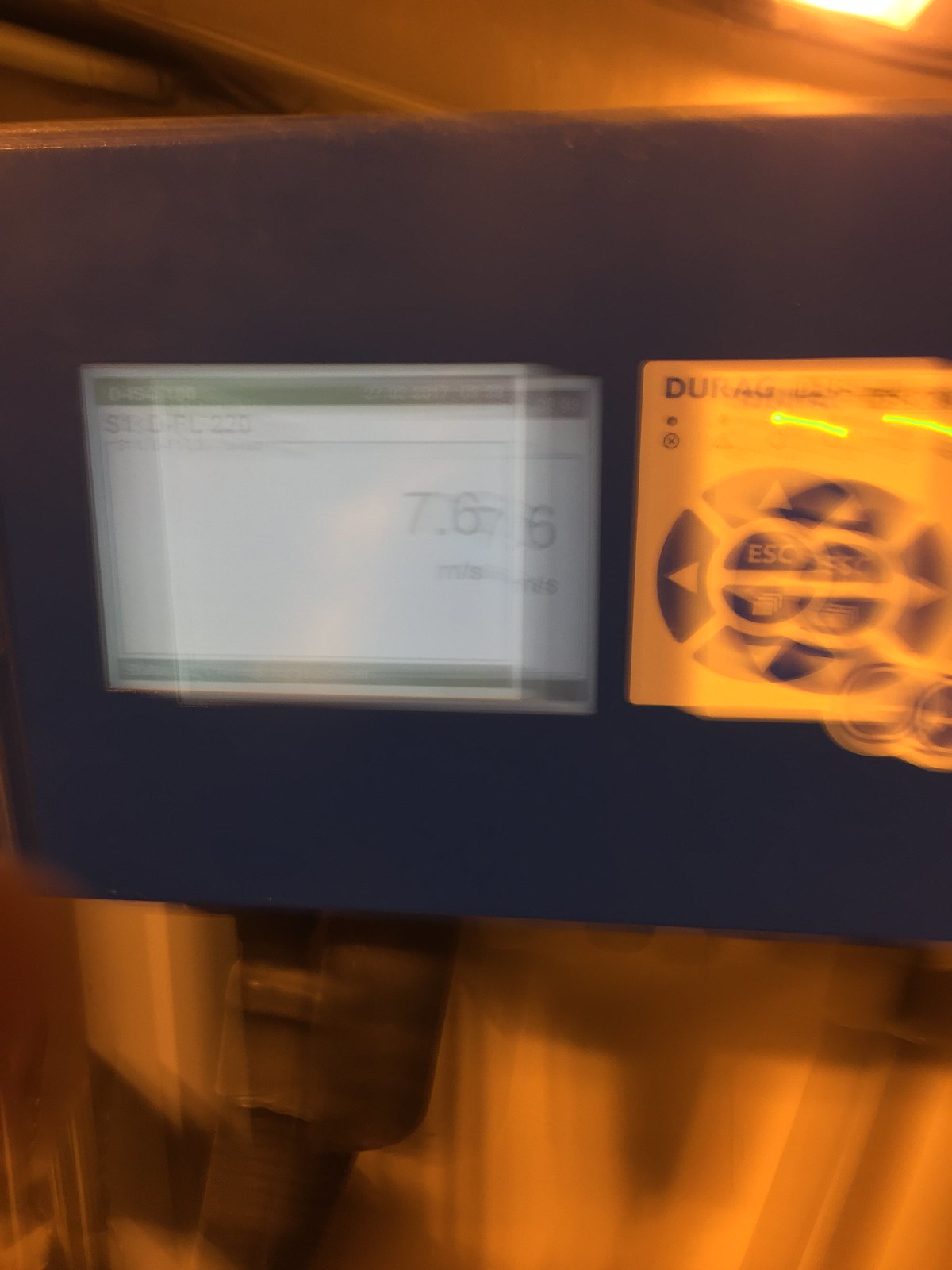This image features a blurry photograph of a digital display, potentially from a screen or a set of signs on a retail shelf. On the left-hand side, there is a white sign with a green header and footer. The header includes the code "D45" followed by some indistinct numbers. The sign also displays two different prices: a lower price of "7.6" and a higher price of "27.02" at the top. The text and details are somewhat unclear due to the blurriness of the image.